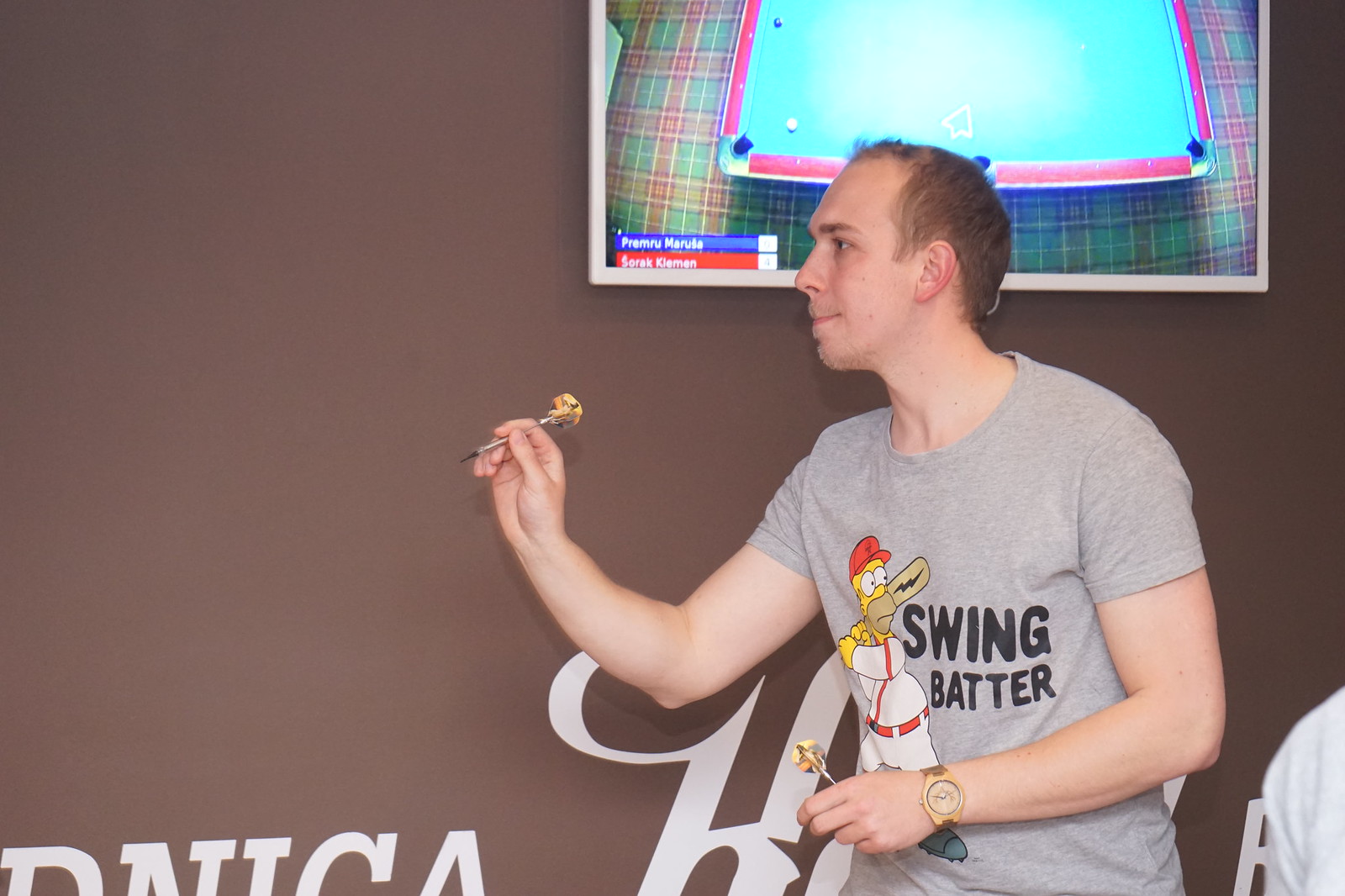A young white man with a fair complexion and short, thinning light brown hair stands near a brown wall, poised to throw a dart with his right hand. He has slight stubble on his chin and is holding another dart in his left hand. He wears a gray t-shirt featuring an image of Homer Simpson in a baseball uniform with a red cap, a white outfit with red accents, holding a baseball bat, alongside the text "Swing Batter." On his right wrist, he sports a golden watch. Mounted on the wall to his right, a gray flat-screen TV displays a live feed of a professional pool game, showing a top-down view of a pool table with some balls on it.